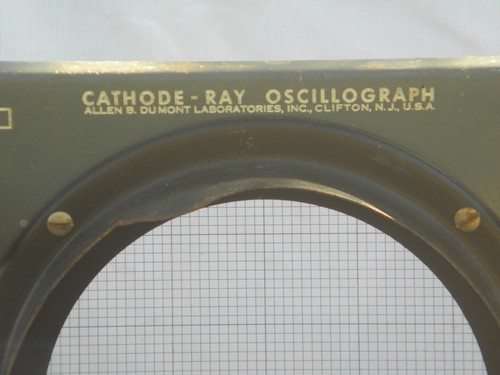The image captures a detailed close-up of a vintage cathode ray oscillograph. The top section showcases a flat, dark green or olive drab painted surface with golden, uppercase text that reads "Cathode Ray Oscillograph, Allen B. Dumont Laboratories, Incorporated, Clifton, New Jersey, USA." Directly below this text is an upper arc of a circular screen resembling graph paper with black crisscrossing lines, housed within a black metal frame. The frame is secured on either side by two brass flathead screws. The background at the very top of the image is a nondescript white or light gray. The photograph focuses on the upper half of the oscillograph, with the lower part and sides truncated, emphasizing the intricate details and design elements of this antique electrical measuring instrument.